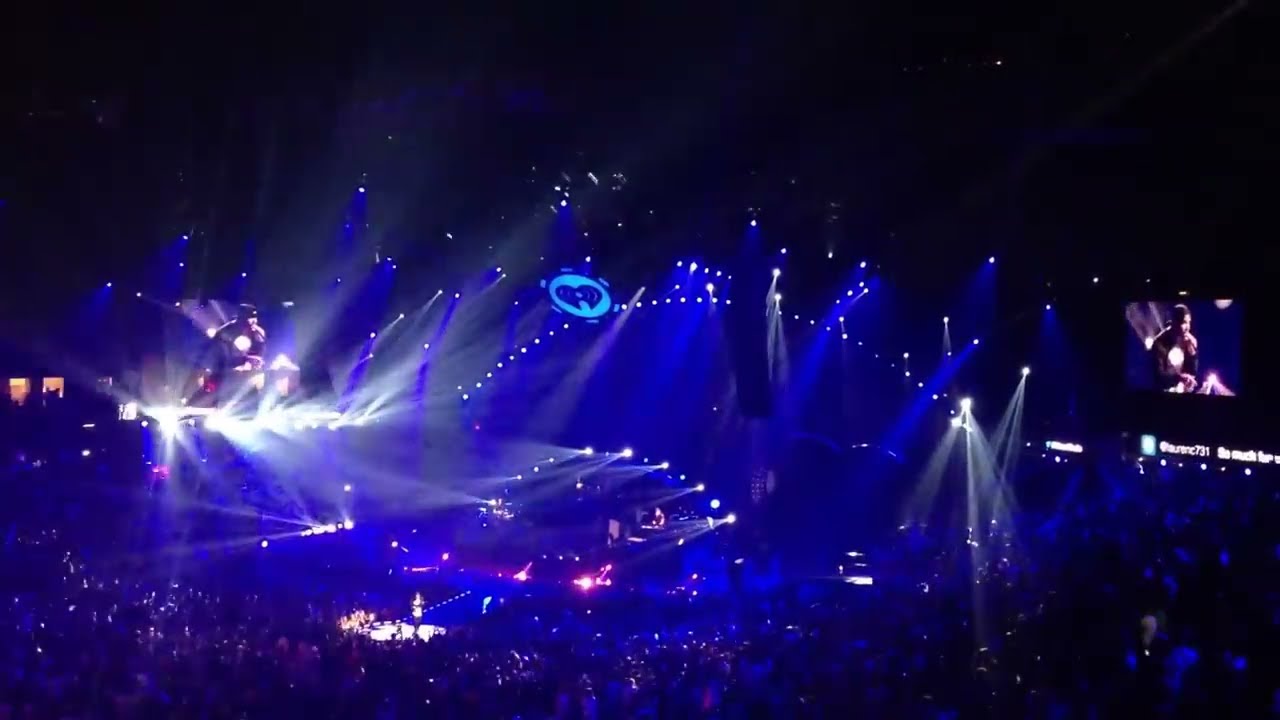This image captures an expansive concert in a massive indoor stadium, pulsating with energy. The photograph, taken from a high vantage point akin to the Nosebleed section, offers a panoramic view of an ocean of glowing blue audience members, with the dense crowd illuminated by waves of blue and white lights emanating from above. At the heart of the concert, the small stage is flanked by enormous screens on either side, displaying a close-up of the lone performer—a figure wearing a hat and engaged with a microphone, likely a singer or rapper. The stage itself features a distinct white spotlight on the performer, contrasting against the predominantly deep blue hue that bathes the scene. Additional arcs of lights, one lower on the stage and another high above, add to the mesmerizing visual spectacle. A notable detail is the small heart emblem, possibly indicating an iHeartRadio event, serving as a focal point amidst the sea of lights and crowd, embodying the grand scale and electrifying atmosphere of the concert.